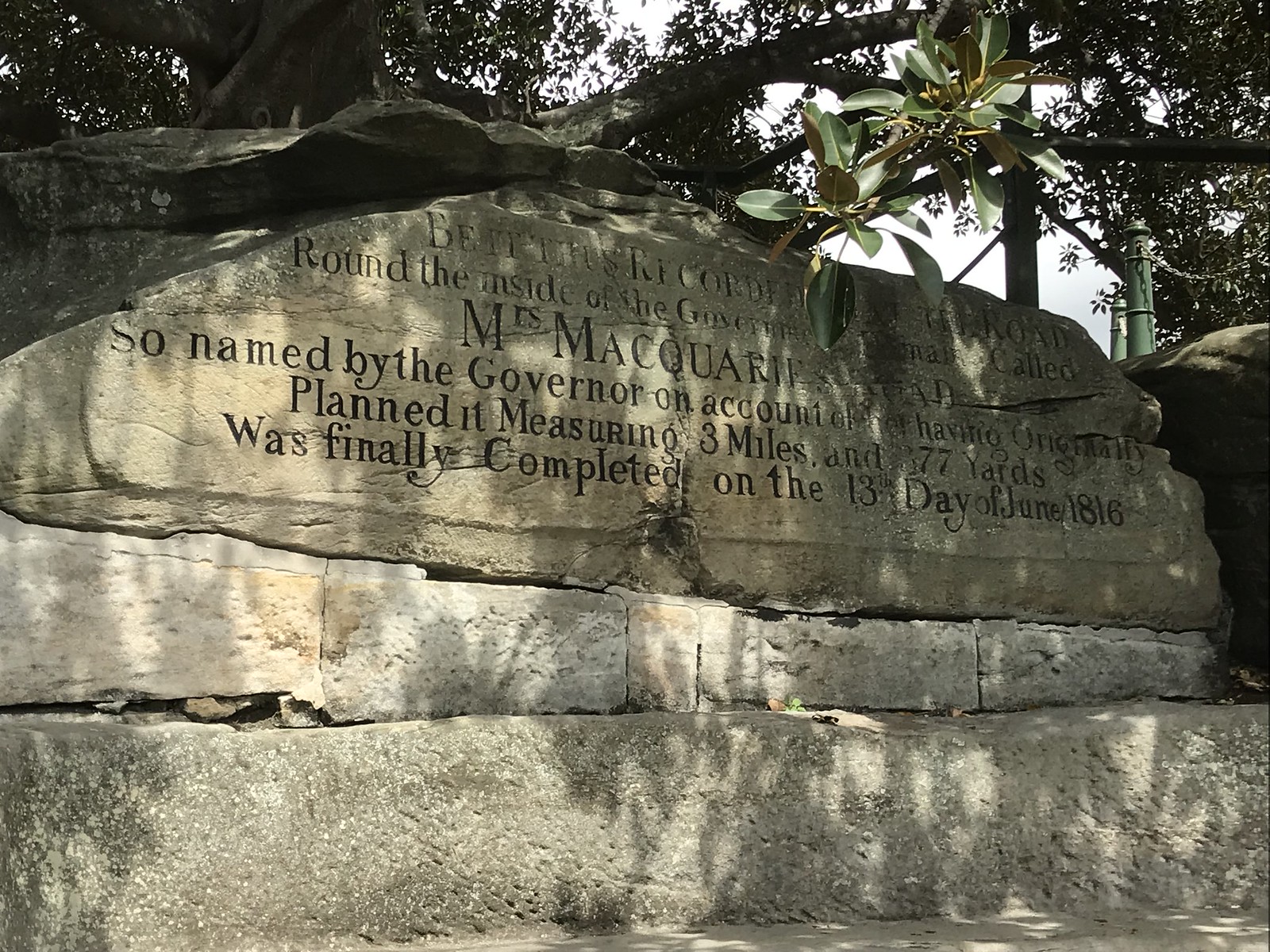The image depicts a large memorial stone embedded in a long, concrete wall with an overhanging tree casting shadows on it. The stone, weighing several tons, has text intricately carved into its surface. Although some parts of the text are difficult to decipher, portions of the engraving can be read. The text mentions, "so named by the governor on account of something planned, it measuring three miles and 77 years was finally completed on the 13th day of June 1816." Additionally, the name "Mrs. McCariff" is visible among the inscriptions. In the background, there is a scenic view of the sky framed by surrounding trees. There is also a smaller, flat stone resting atop the larger memorial stone.